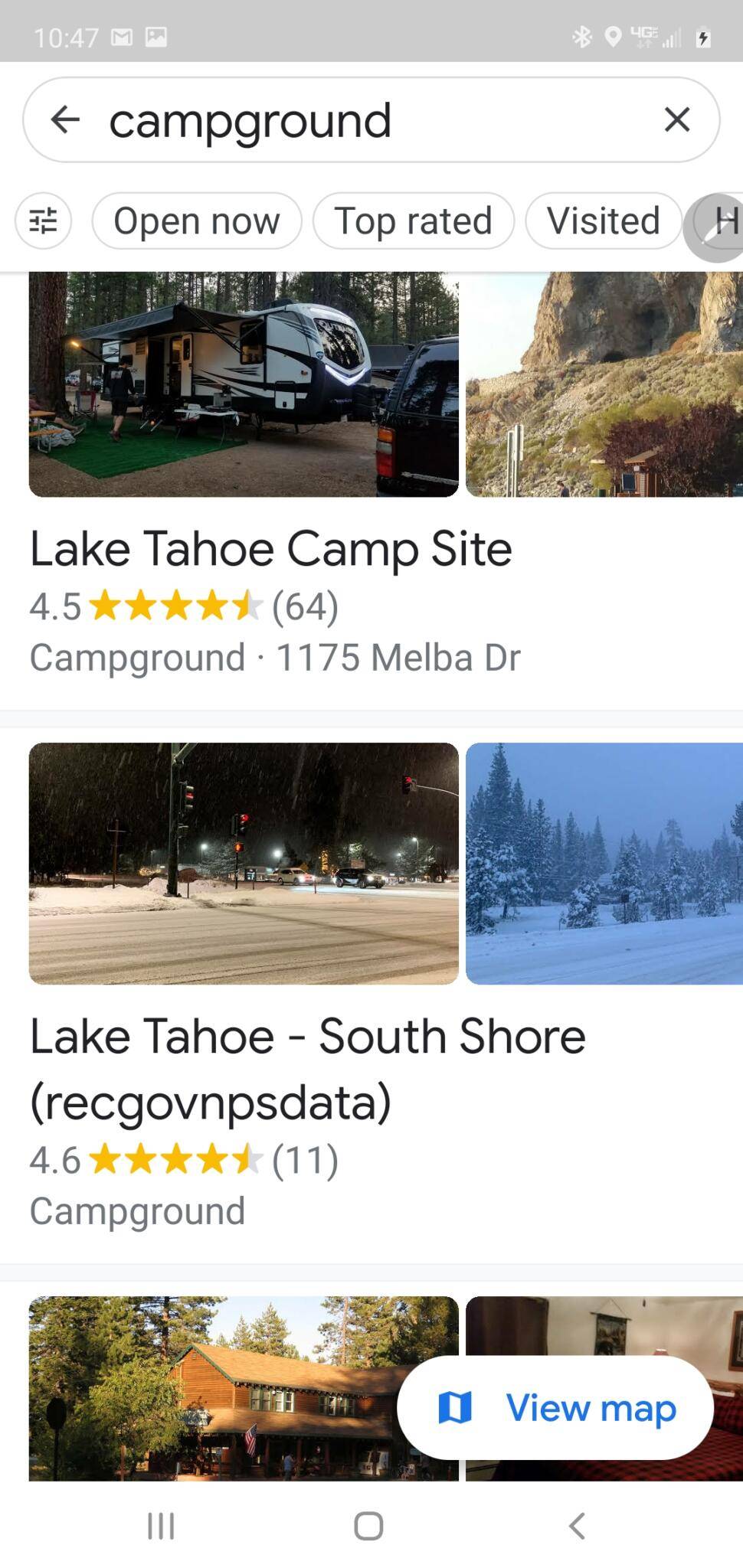**Detailed Image Description:**

The image is a screenshot from a smartphone or tablet, presenting a detailed display of a campground search or review platform. 

At the top of the device's screen, there is a dark gray bezel displaying the time as 10:47 without specifying AM or PM. The status bar includes several icons: the Gmail symbol (an envelope inside a circle), an image icon (a square with white mountains and a white sun or sky), the Bluetooth symbol, a GPS pin symbol, the 5G network indicator showing three out of five bars, a signal strength indicator with three out of five bars, and a battery symbol with a black lightning bolt inside it, indicating the device is being charged.

Below the status bar, there is a navigation section with an oval shape containing a black left arrow, the word “Campground” in black text, and a black right arrow. This section suggests navigation within the app or website.

The main content comprises multiple interactive buttons and detailed descriptions:

1. **Filter Button**: A circular button with three horizontal lines intersected by a vertical line, iconographically representing sliders for filters or settings.
   
2. **Oval Buttons**: Four oval buttons with black text, labeled “Open Now,” “Top Rated,” “Visited,” and one partially visible button starting with “H.”

3. **Pen Shortcut**: A translucent dark gray circle with a white pencil icon, indicating the presence of a stylus or note-taking feature on the device.

The content also includes detailed listings of campgrounds:

- **First Listing**: 
  - Image: A white camper with black stripes against a backdrop of tan, yellow, and brown mountains.
  - Title: "Lake Tahoe Campsite"
  - Review: 4 out of 5 stars with 64 reviews
  - Category: "Campground"
  - Address: "1175 Melba Dr."
  - Description: A snow-covered road with black poles.
  
- **Second Listing**:
  - Header: “Lake Tahoe - South Shore” with “Record Governance Data” in parentheses.
  - Review: 4.6 out of 5 stars with 11 reviews
  - Category: "Campground"
  - Description: Snow-covered road lined with snow-covered evergreen trees.

- **Third Listing**:
  - Image: A log cabin with a tan roof.
  - Interactive Button: Floating off-gray oval button labeled “View Map,” with a map icon depicted in dark blue and white.

Additional visual elements include three black lines, a black circular icon, and a left-pointing black arrow, which might be part of the app's interface or design.

Overall, the image showcases a comprehensive view of a campground review or search platform on a mobile device, providing users with filter options, detailed reviews, and interactive buttons for further actions.